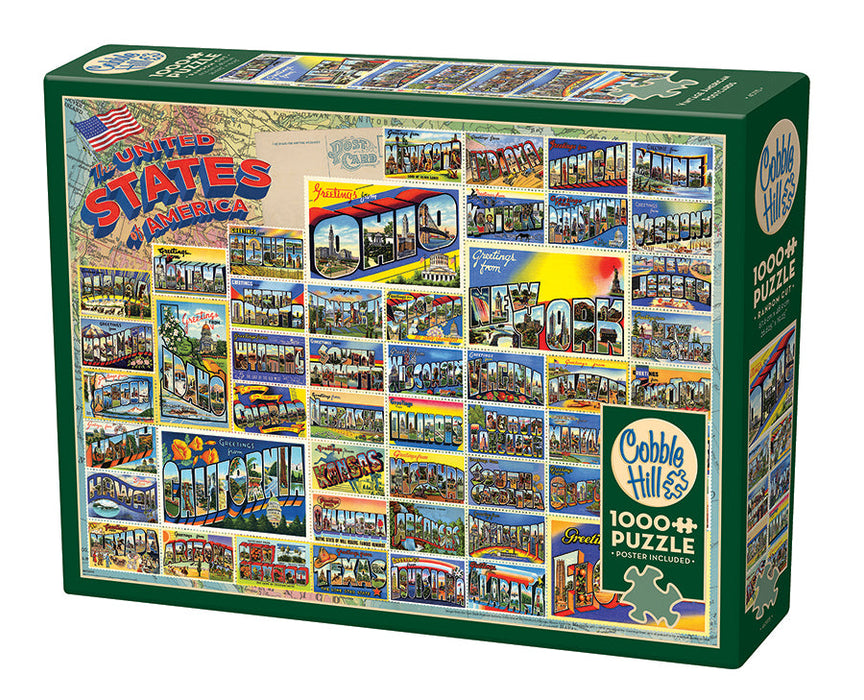The image depicted is a color photograph in landscape orientation, showcasing a puzzle box at an angle, with the top of the box facing the viewer and part of the right panel visible. The box is designed to represent a 1000-piece puzzle of the United States of America. Dominating the top left corner is a waving U.S. flag, accompanied by the words "United States of America" in red with a blue drop shadow, giving it a 3D effect. This title is set on a curved backdrop.

The box cover features a vibrant display of individual square illustrations, each representing a different state with pop art visuals of notable items associated with each state. Arranged in multiple rows, these illustrations collectively highlight all 50 states. Adding to the detailed design, the lower right segment of the box includes a dark green rectangle with a cream-colored circular logo. Inside the logo appears a blue-outlined puzzle piece and the brand name "Cobble Hill" in light blue lettering, along with the phrase "1000 Piece Puzzle" and an indication that a poster is included.